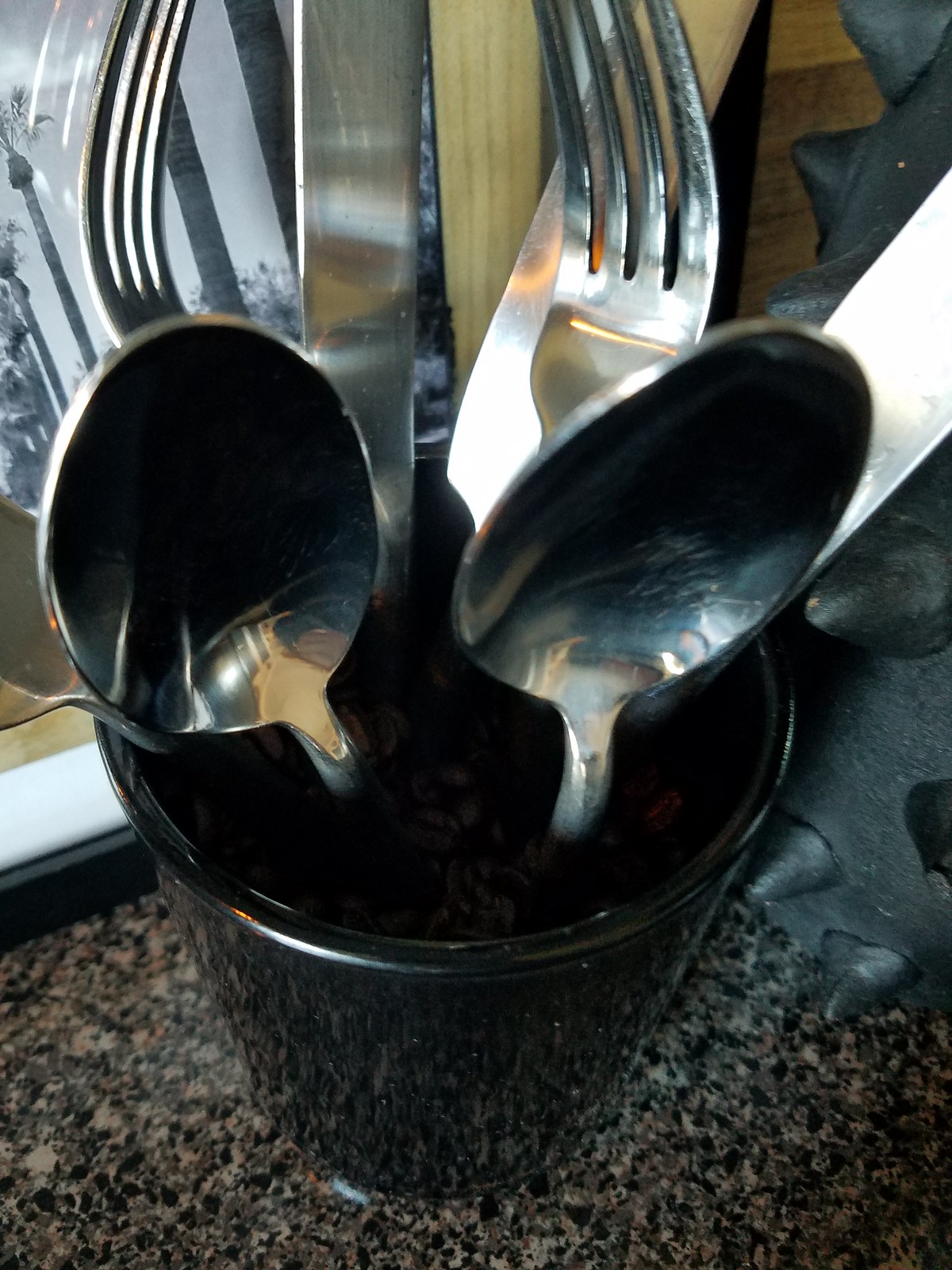The image captures a close-up view of a black, smooth, and shiny cup, possibly made of plastic or ceramic, containing an assortment of silverware. Inside the cup, there are two forks, two spoons, and three butter knives, all made of stainless steel with some visible scratches, suggesting they have been used. The forks have four tines and the spoons are large, not teaspoons. The cup is positioned on a countertop with a marbled pattern in shades of beige, black, and gray. In the background, there is a light-colored walnut wooden window frame and what appears to be a black-and-white framed picture or window, possibly showing trees. To the right of the cup, there is another kitchen gadget with spikes, likely a black rubber or soft material. The overall setting seems to be a kitchen, with various indistinct decorations in the background.